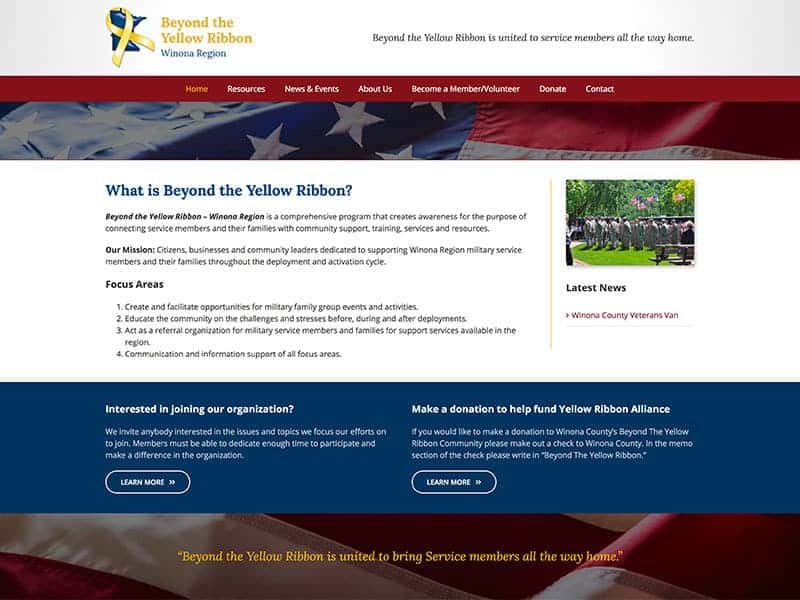The image is a detailed webpage for the organization "Beyond the Yellow Ribbon," specifically for the Winona Region. The layout is predominantly wider than it is tall, designed to fit a large computer screen. At the topmost section, there's a gray banner featuring the organization's logo—a blue emblem encircled by a yellow ribbon. Adjacent to the logo, the text "Beyond the Yellow Ribbon, Winona Region" is prominently displayed, with "Winona" carefully spelled out for clarity. On the right side of this banner, a tagline reads, "Beyond the Yellow Ribbon is united to service members all the way home."

Beneath this banner, there's a distinguishing red menu bar, resembling a taskbar, followed by an image of the American flag positioned as a rectangular element. Centered on the page is an informative section introduced by the blue headline, "What is Beyond the Yellow Ribbon? Let's find out."

The body text explains that Beyond the Yellow Ribbon, Winona Region, is a comprehensive program aimed at raising awareness to connect service members and their families with community support, training, services, and resources. The mission of the organization highlights several focus areas such as organizing military family events, educating the community about the experiences of returning soldiers, assisting with the reintegration of soldiers into civilian life, and providing ongoing communication and support.

The webpage further offers options for visitors to join the organization or make a donation. Emphasizing the challenging nature of transitioning from a war zone to civilian life, the overarching goal of Beyond the Yellow Ribbon becomes evident: to aid service members in their return home.